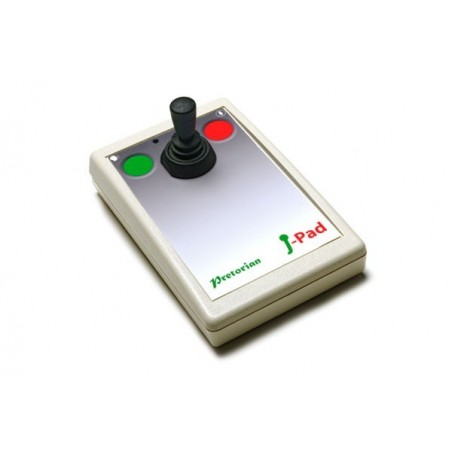This image shows a detailed, photoshopped PNG depiction of a control device labeled "Praetorian J-Pad" with light shadowing and a white, transparent background. The device is a rectangular, off-white plastic joystick controller measuring approximately 2-3 inches in width and height. It features a distinctive ombre pattern on the surface, transitioning from gray to white. Prominently, the top of the controller houses two circular buttons: a green button on the left and a red button on the right, the latter displaying a downward arrow symbol. Centrally positioned between these buttons is a black joystick lever. The words "Praetorian" and "J-Pad" are inscribed in green and black text near the bottom of the controller. The image is notable for its simplicity, with no borders or other identifiable elements besides the device and its shadow.